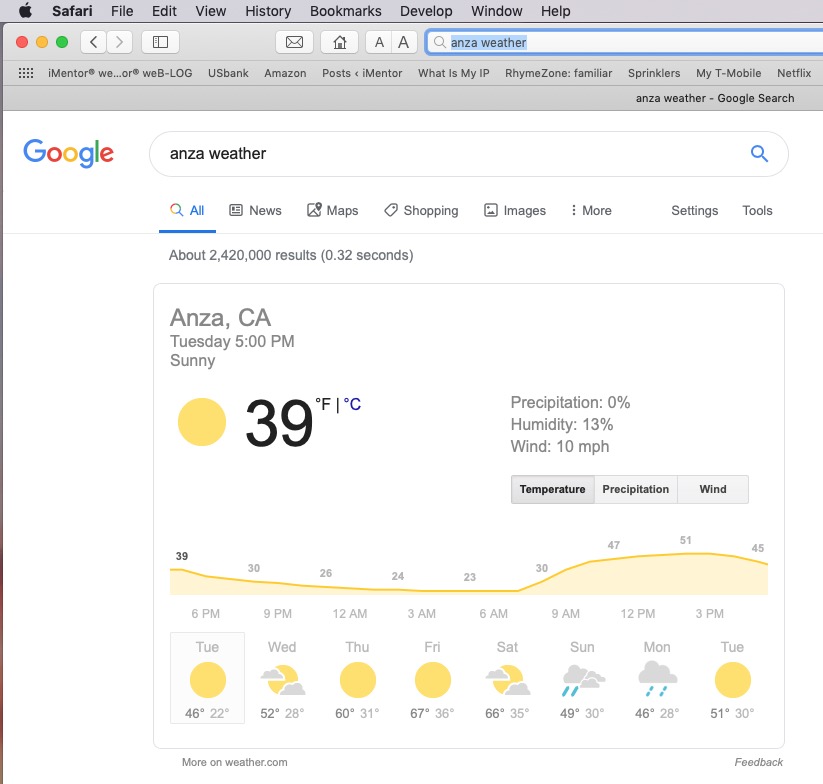This screenshot captures a user searching for "ARANZA weather" on the Safari browser, specifically using the Google search engine. The results are displayed under the "All" tab, where a prominent weather information box from Weather.com appears at the top. This box details the current weather conditions in Anza, California, as of Tuesday at 5 p.m. The weather is described as sunny with a temperature of 39°C, with the 'C' for Celsius highlighted in blue. Additional weather details include 0% precipitation, 13% humidity, and wind speeds of 10 miles per hour. A graph also illustrates the temperature trends from 6 p.m. on Tuesday to 3 p.m. the next day, giving a comprehensive view of the local weather forecast.